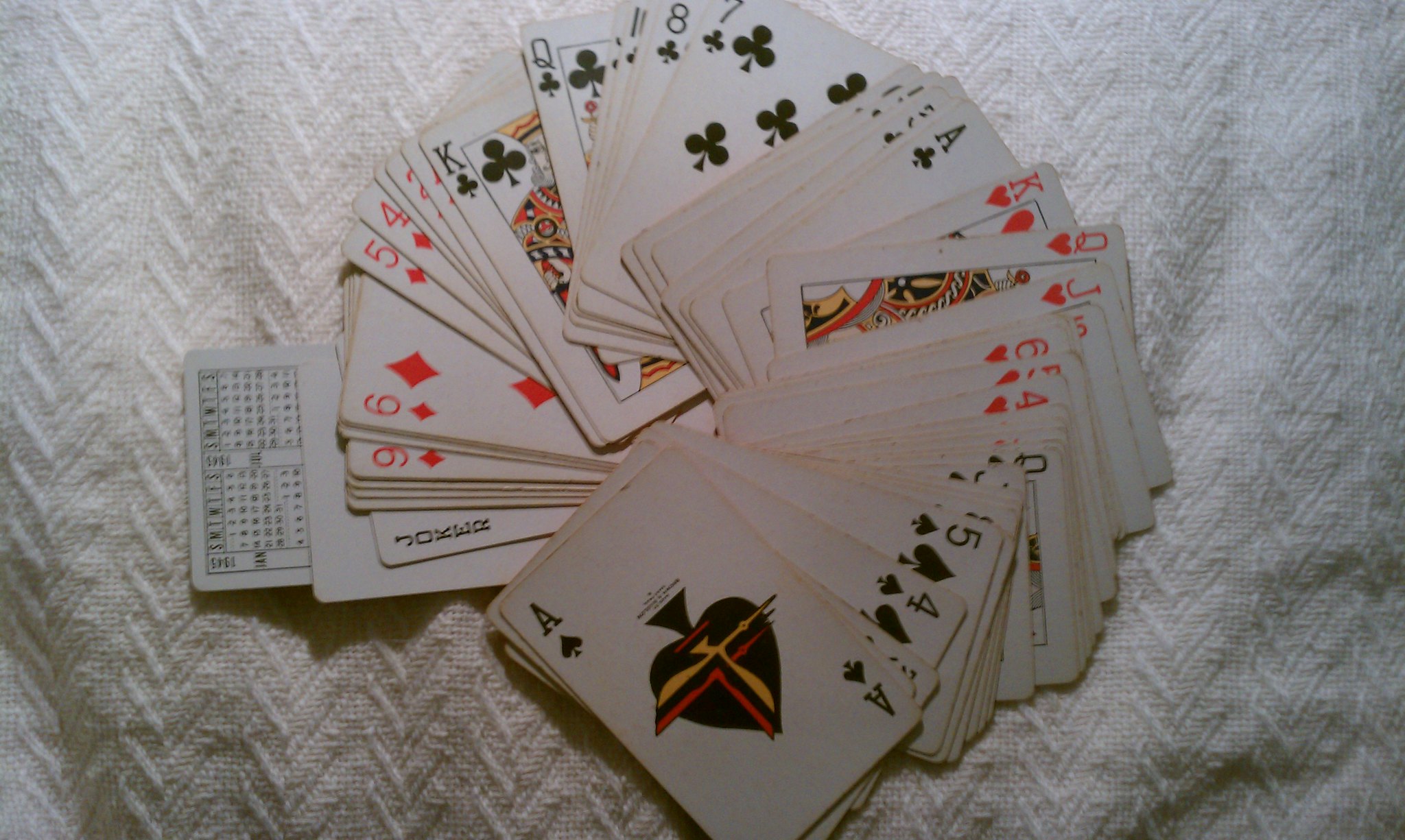This image showcases a scattered assembly of playing cards spread across a textured white fabric, likely a towel or blanket. The cards form an irregular semi-circle, some partially overlapping others in a casual, unorganized manner. Among the visible cards, a variety of suits can be identified, including clubs, diamonds, hearts, and spades. Noteworthy cards within the array include the King of Clubs and the Queen of Diamonds, alongside a range of cards from aces to numerical values. Dominating the foreground is an Ace of Spades, adorned with a distinctive black and red graphic design, standing out against the traditional card designs. An index card, potentially a scorecard or reference guide, with numbers and text, is also visible, suggesting its relevance to the game or deck. The haphazard arrangement implies that the cards might have been casually discarded following a game or purposefully laid out for selection in an informal card-playing scenario.